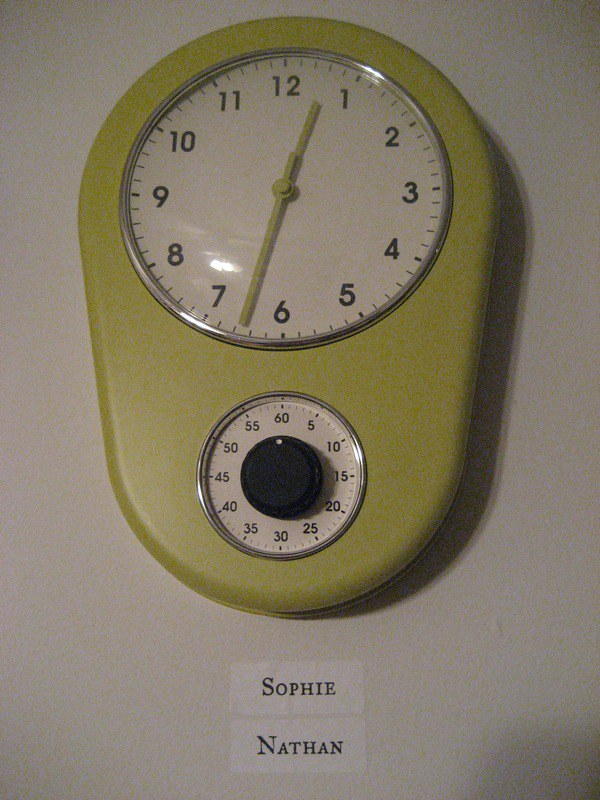This photo features an old-fashioned, yellow metallic clock and timer combination mounted on a plain, white wall. The uniquely shaped clock is an oval that narrows at the bottom. The upper part of the device houses a larger round white clock face encircled by a silver band. The clock displays black Arabic numerals from 1 to 12, with yellow hands indicating the time at 12:32. Below the clock face, a smaller dial functions as a timer, with numbers ranging from 5 to 60 in five-minute increments, and individual hash marks for each minute. The timer includes a central black knob with a white dot showing its current setting. The names "Sophie and Nathan" are visible beneath the clock, printed on the wall.